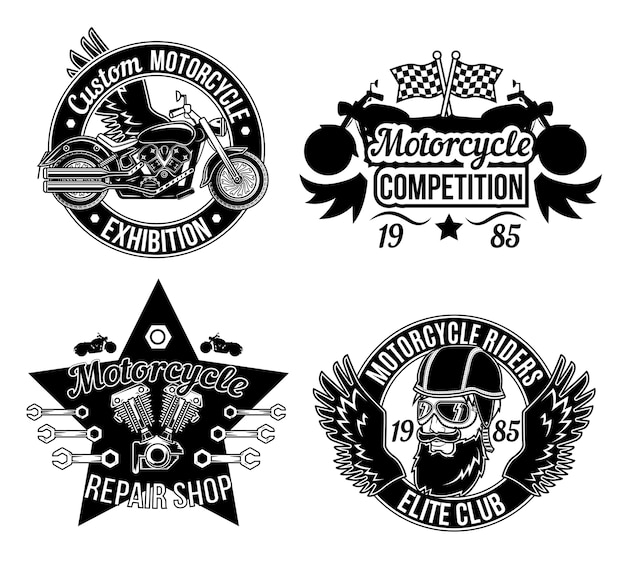This image comprises four distinct black-and-white logos set against a white background, each representing different aspects of motorcycle culture. The top left logo is a circular emblem with a black ring and white text that reads "Custom Motorcycle Exhibition." Inside, it features a detailed illustration of a motorcycle with wings extending from the sides. Moving to the top right, another black and white logo displays two checkered flags crossed above the mirrored silhouettes of two motorcycles. This emblem bears the text "Motorcycle Competition" and the year "1985."

In the bottom left corner is a five-pointed black star encapsulating various elements: a motorcycle engine in the center, surrounded by the silhouettes of six wrenches—three on each side. Above the left and right arms of the star are two motorcycles, with a lug nut situated at the top point of the star. This logo is marked with the words "Motorcycle Repair Shop." Lastly, the bottom right logo is also circular with a black ring and white lettering stating "Motorcycle Riders Elite Club." It features bold black wings flanking each side of the circle and, at its center, a bearded man wearing a motorcycle helmet and goggles. The year "1985" is split on either side of his face in black text.